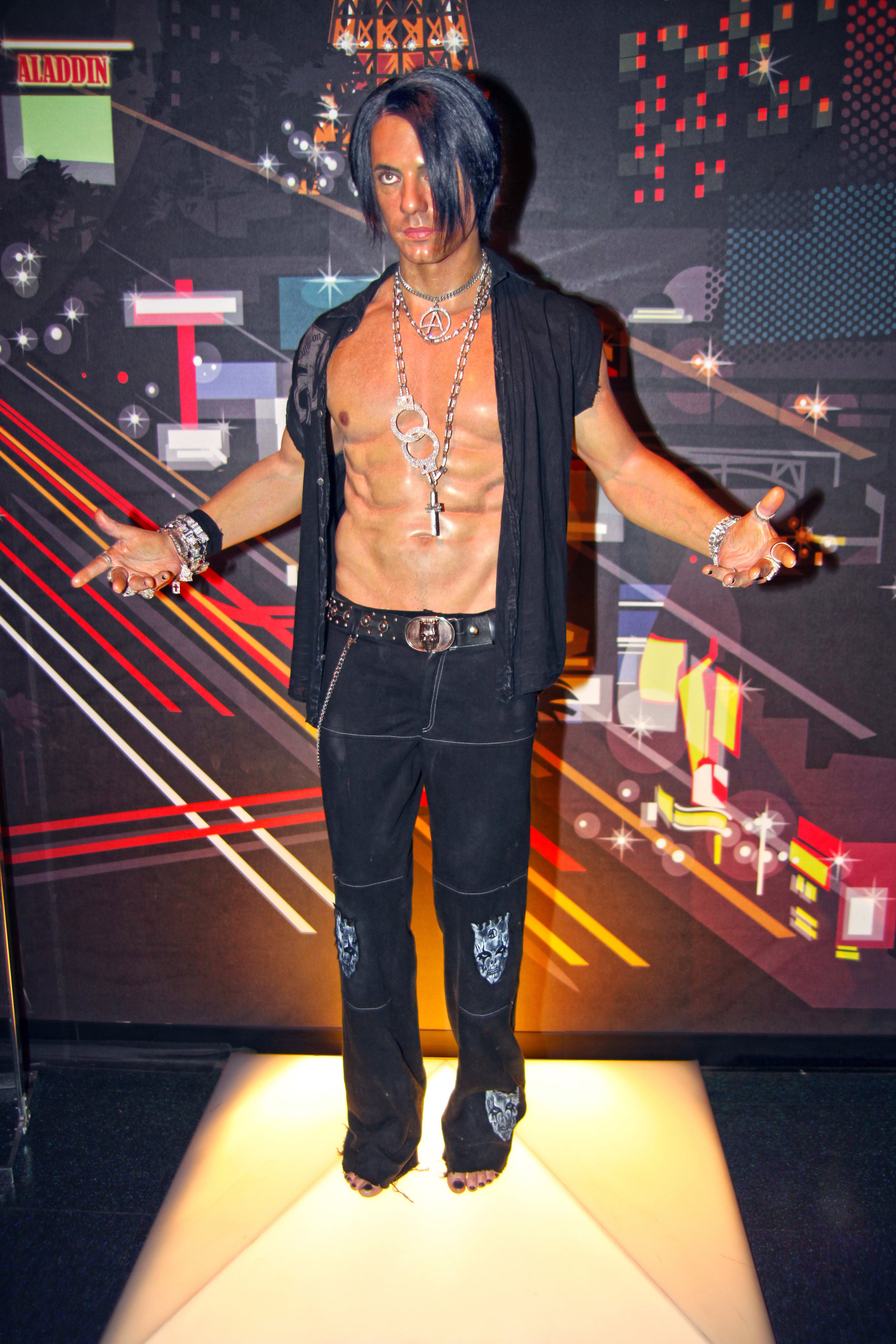In this picture, a well-built man stands on a stage, posing confidently toward the camera. He has long, straight, ironed black hair that cascades over his left eye and down to his chin. His muscular physique is prominently displayed, as he wears an open black vest that reveals his chiseled abdomen and chest. Around his neck, he sports multiple chains, both long and short, and his wrists are adorned with numerous pieces of jewelry. His outfit is completed by a pair of black jeans, cinched by a belt with a brown buckle.

The stage beneath him has a striking design, predominantly white in the center, suggesting a spotlight beaming down on him, while the outer edges are shrouded in black. Behind him, a detailed backdrop adds depth to the scene. The backdrop features diagonal stripes that resemble beams of light descending from above, alongside city-like decorations with windows illuminated in red lights. The upper left corner of the backdrop prominently displays the word "ALADDIN" in small, red uppercase letters. The overall setting has a cartoonish vibe, with various colored lines indicating different speeds, creating a dynamic and vibrant atmosphere.